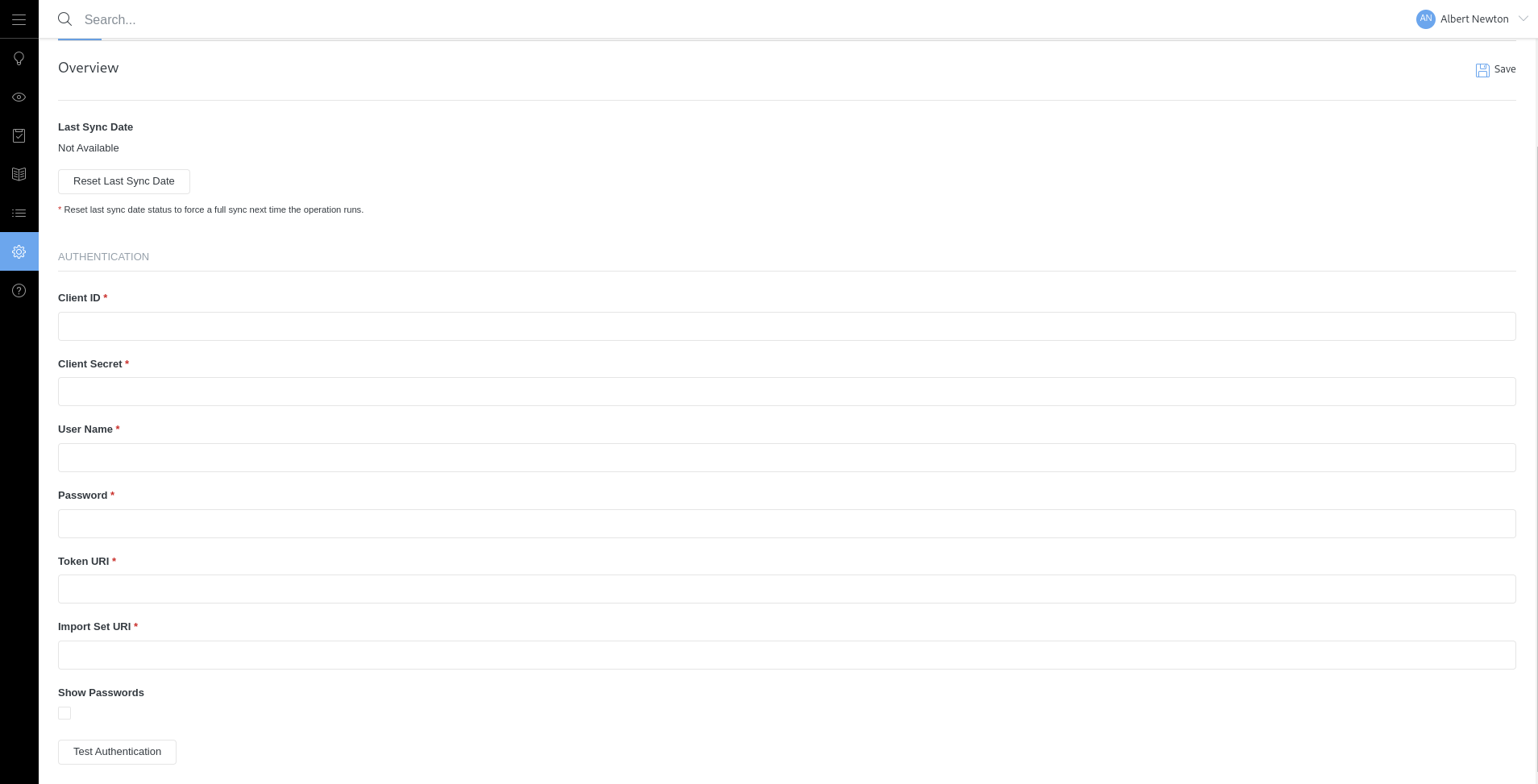The image depicts an overview page of a software interface. At the top left corner, there is a labeled "Search" bar. Below the search bar, there is a section titled "Overview," followed by "Last Sync Data," and an option to "Reset Last Sync Data." There are several text boxes or fields displayed on the page, including fields for "Client ID," "Username," "Password," and a field for a URL. The overall layout appears structured to manage synchronization settings and user credentials efficiently.